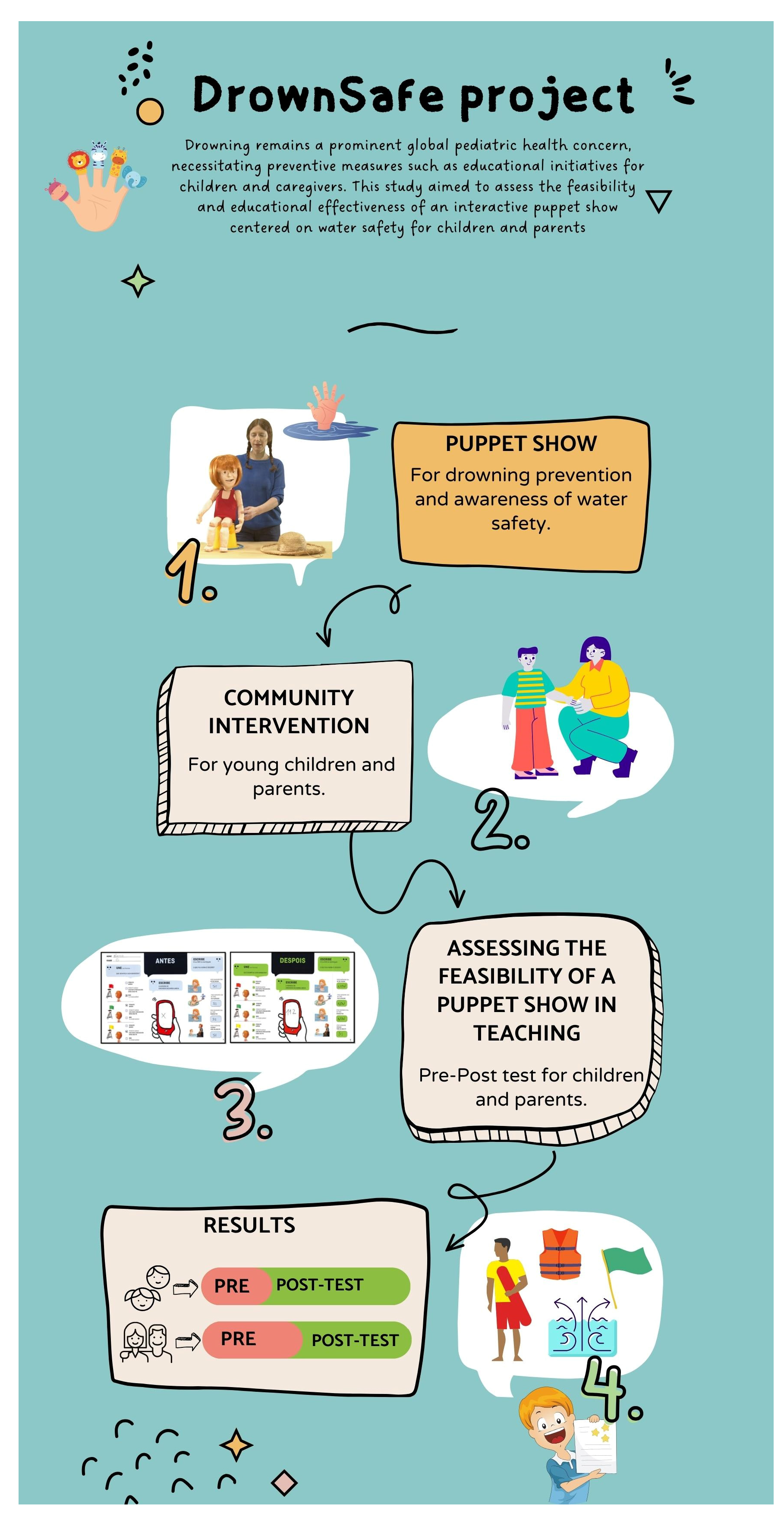The poster titled "Drown Safe Project" is a detailed, educational visual aid designed to address the global pediatric health concern of drowning. It advocates for necessary prevention measures through educational initiatives targeting children and caregivers. The primary color scheme encompasses a vibrant palette, featuring reds, whites, blues, yellows, blue-greens, oranges, blacks, and pinks, with a predominant greenish-blue background.

At the top, in large black print, the title "Drown Safe Project" is prominently displayed, followed by a smaller subtitle that explains the urgency of the issue: "Drowning Remains a Prominent Global Pediatric Health Concern, Necessitating Preventive Measures, such as Educational Initiatives for Children and Caregivers." The poster introduces an interactive puppet show as a fun and effective way to teach water safety.

To the left of the main text, there's an illustration of a hand with finger puppets featuring a jester, a lion, a giraffe, a zebra, and an elephant. This is followed by the first section of the poster detailing the program's steps. Labeled as number one, it depicts a woman using a puppet, accompanied by a speech bubble. To the right, an orange rectangle with black print states "Puppet Show for Drowning Prevention and Awareness of Water Safety," leading into a gray rectangle marked "Community Intervention for Young Children and Parents."

The second step, labeled with a number two, appears to the right. It shows an adult kneeling to speak to a child within a white speech bubble, with a gray rectangle below it, stating "Assessing the Feasibility of a Puppet Show in Teaching Pre-Post Test for Children and Parents." Nearby, another speech bubble in Spanish indicates "antes" and "después" for before and after.

In the bottom left corner, a brownish-gray rectangle labeled "Results" includes images of children and adults with "Pre" and "Post Test" results depicted in pink and green backgrounds respectively. Lastly, the poster's fourth and concluding section shows a child holding a piece of paper with a speech bubble illustrating a lifeguard, a life vest, a green flag, and a riptide, emphasizing the educational content imparted through the program.